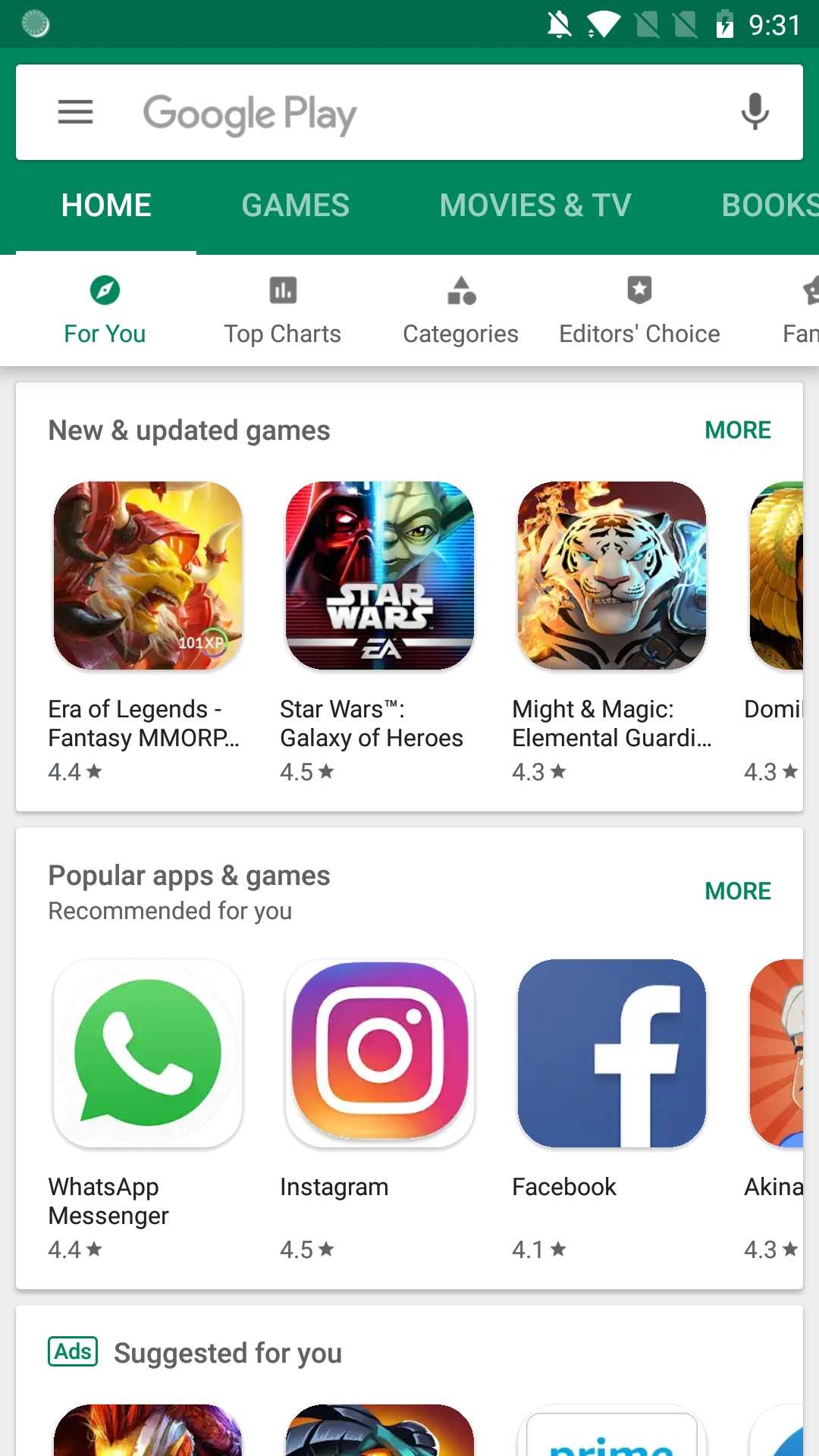The image is a screenshot taken on a smartphone, displaying the Google Play Store interface. At the top edge of the screenshot, the phone's status bar features a green background with various indicators: a silent bell icon, a Wi-Fi network logo, a partial battery bar, and the time "9:01," all in white color.

Below the status bar, the header of the Play Store is visible, showcasing a search bar with three horizontal lines for options, the words "Google Play" written in gray ink, and a microphone icon for voice search. The main navigation tabs are listed horizontally: "Home," "Games," "Movies & TV," and "Books." Additional navigation options, "For You," "Top Charts," "Categories," and "Editor's Choice," are also present, with "For You" highlighted in green ink.

The primary content of the screenshot focuses on various sections within the Play Store. There is a section for "New and Updated Games," displaying various game icons, followed by another section labeled "Popular Apps & Games," which includes well-known applications like WhatsApp, Instagram, and Facebook, highlighted under "Recommended for You."